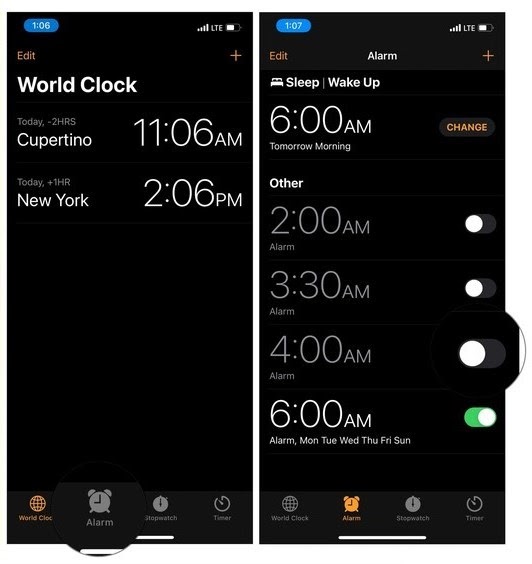The image consists of two smartphone screenshots displayed side-by-side. The screenshot on the left shows a screen with the time highlighted as 1:06 PM in a blue box. The screen includes sections labeled "Edit," "World Clock," and "Today." The World Clock section lists Cupertino with a time of 11:06 AM and New York with a time of 2:06 PM. Below this, there is an orange globe icon labeled "World Clock." Additionally, the screen features icons for "Alarm," "Stopwatch," and "Timer."

The screenshot on the right displays a screen with the time shown as 1:07 PM. This screen offers options such as "Edit," "Alarm," and "Sleep." It specifies a "Wake up" time of 6:00 AM for the next morning, with an orange hyperlink labeled "Change." Under the "Other" section, there are alarms set for 2:00 AM, 3:30 AM, 4:00 AM, and 6:00 AM.